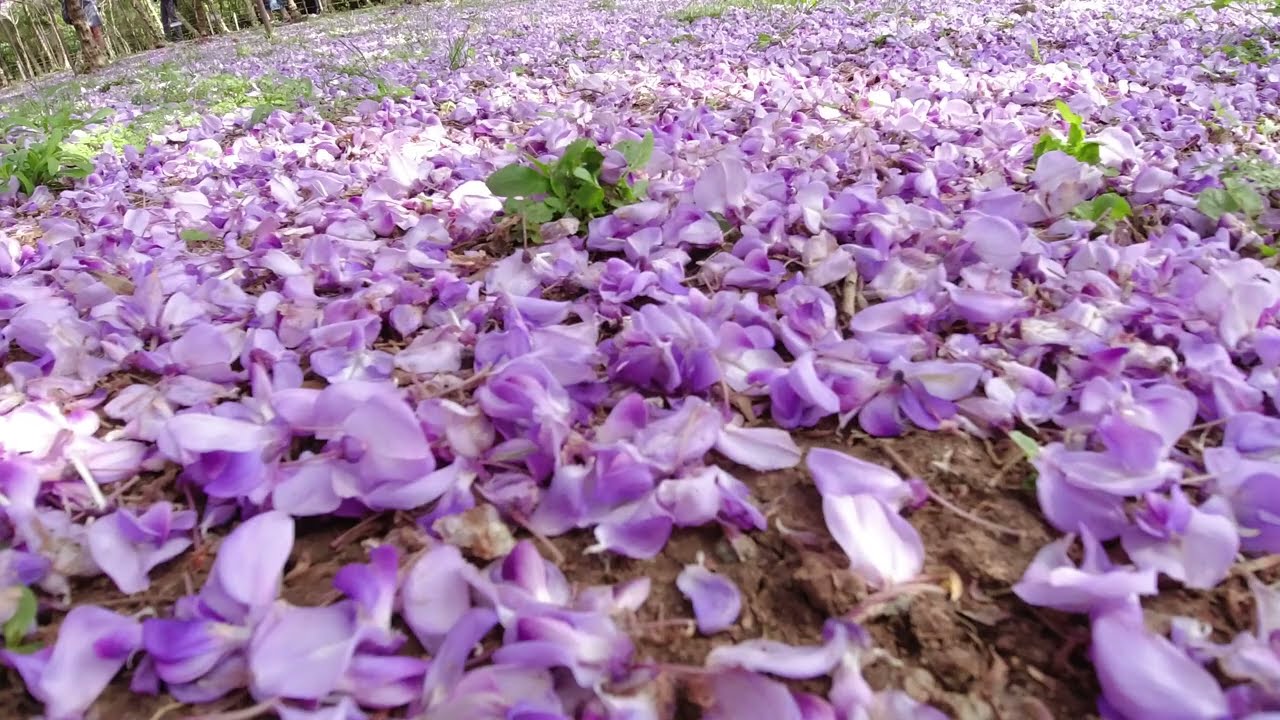The image depicts a close-up view of a field blanketed by small, lilac-colored flower petals, possibly from magnolia trees. These delicate petals, varying in shades of purple, intermingle with patches of green plants and weeds, especially notable in the top third and left side of the picture. The lush field extends toward the horizon, with a subtle dappled sunlight illuminating parts of the scene, creating an interplay of light and shadows. In the bottom right corner, the brown earth peeks through the carpet of petals, while the top left corner features a sliver of trees with diverse trunks and foliage, adding depth to this serene, pastoral landscape.